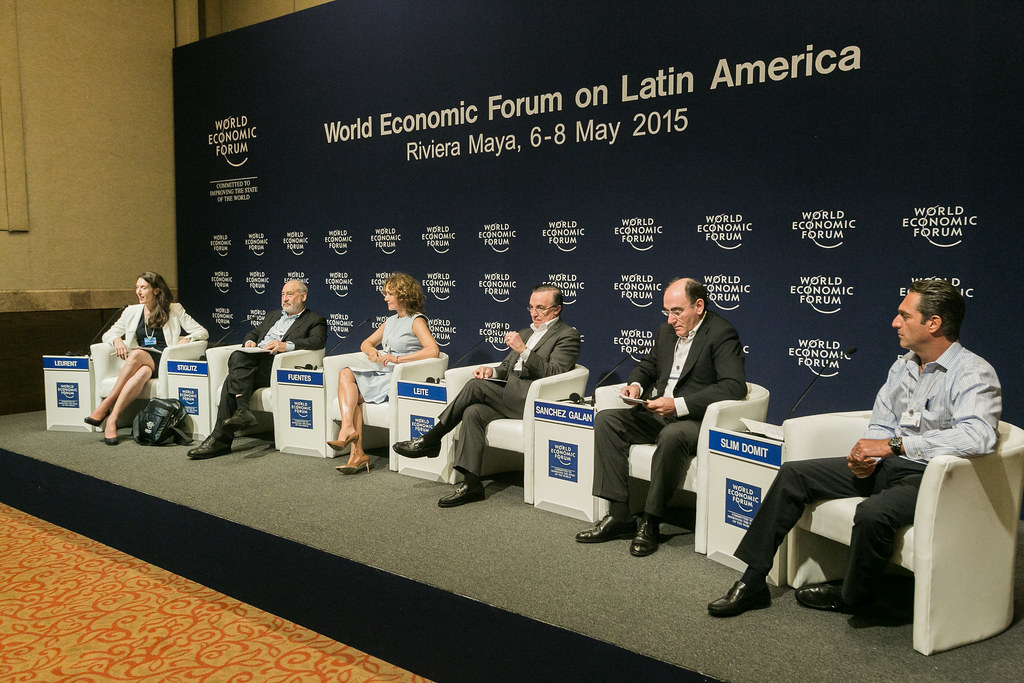The image depicts a formal meeting at the World Economic Forum on Latin America held from May 6-8, 2015, in Riviera Maya. Six individuals, consisting of two women and four men, are seated on a narrow stage in semicircle-shaped white leather chairs with low backs. Each person is positioned next to a small side table, which holds a microphone and name plaque with blue tags indicating their names or possibly their origins. Behind them is a large blue backdrop prominently displaying the event's name and dates, along with repeated World Economic Forum logos. The participants appear to be dressed formally, with the men in suits and the women in dresses. The first lady, in a black dress with a white sweater, seems to be the one currently speaking. The men mostly wear black shoes, black or gray pants, and suits, except for one man who is dressed in a blue shirt. The overall scene suggests a high-level discussion possibly focused on significant economic or political issues in Latin America.